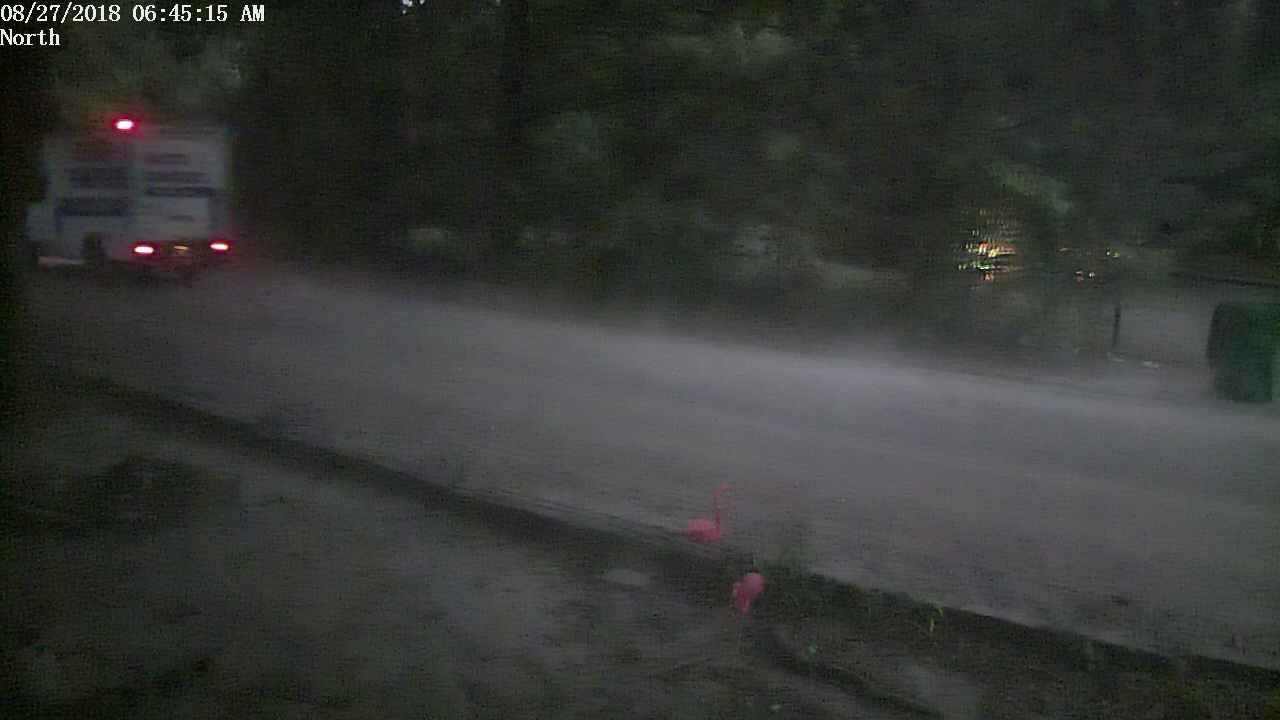This image captures a blurry and grainy street scene, likely taken from a roadside camera or dash cam on August 27, 2018, at 6:45 a.m. The view is directed towards a roadway, bordered by tall trees on the right and a patch of dirt with some green weeds and pink flamingo figures on the left. Dominating the scene is a boxy vehicle, likely an ambulance or a small moving van, characterized by its white color adorned with blue, red, and possibly green stripes. The vehicle's tail lights emit three distinctive red dots, and there's a light illuminating the license plate in yellow. Additionally, a yellow light is seen emanating from behind one of the trees. The timestamp and 'north' direction indicated in the top left corner suggest that this might be a frame from a surveillance or wildlife camera. The overall setting appears to be in the early morning hours, with a somewhat eerie, early dawn atmosphere enveloping the scene.